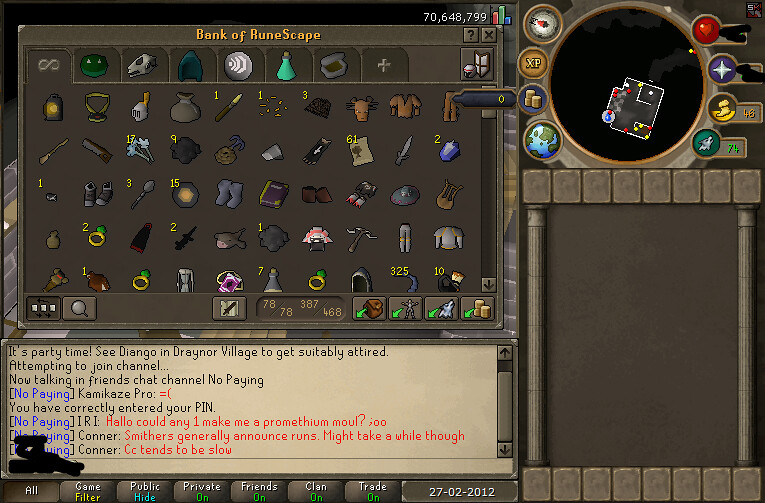This image is a detailed screenshot from the video game RuneScape, specifically displaying the in-game bank interface. Prominently, at the top of the screen, "Bank of RuneScape" is written in bold yellow text within a large gray rectangle that showcases numerous items. These items, laid out in a grid, include pixelated representations of armor, jewelry, boots, clothing, food, tools like a shovel and saw, and various other equipment. Some items have yellow numbers beside them, indicating quantities. In the top-right corner, the screenshot shows a circular black map that marks different locations and features with red and yellow circles, providing a navigational aid.

Below the item grid is a tan chat box with black and red text, where ongoing social interactions are visible. Conversations include phrases like "it's party time, see Jango and Draenor Village to get suitably attired," and other messages detailing attempts to join different chat channels and acknowledging the correct entry of a PIN. This chat box is a key element for player communication. Additionally, the bottom of the screen features several tabs, likely representing different options or functionalities for player interaction and inventory management. The top-left corner of the interface prominently displays a significant number of gold coins—70,648,799—indicating the wealth stored in the player’s bank.